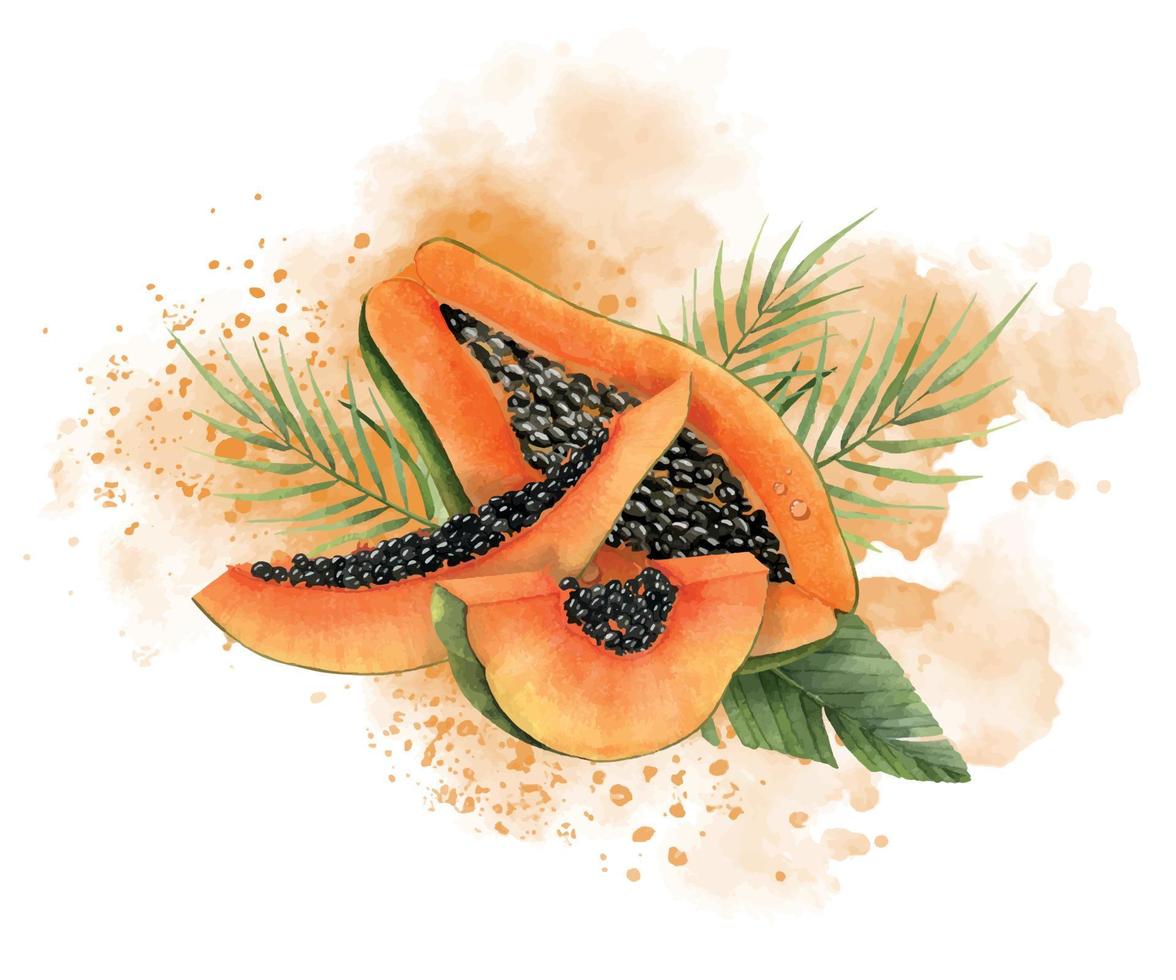This image is an artistic drawing of a papaya that showcases various segments of the fruit laid out on a backdrop of vibrant, painterly splashes of orange and white. The scene is centered around a larger papaya half that is split open to expose its multitude of black seeds. In front of this half, there's a one-fourth slice of the papaya, also showing its seedy interior. Close to these, another piece of papaya, resembling a thick wedge, sits prominently, with the same seed-filled core. The papayas rest on a bed of diverse green leaves, including a notably large palm leaf and several skinnier variants. The overall composition is accentuated by a solid white background, enhancing the vivid orange hues of the papaya and the contrasting greens of the leaves. Tiny brown speckles are scattered around the fruit pieces, adding texture to the image. The close-up perspective allows a detailed view of the fruit, making visible even the small white dots like water droplets on the flesh of the papaya.